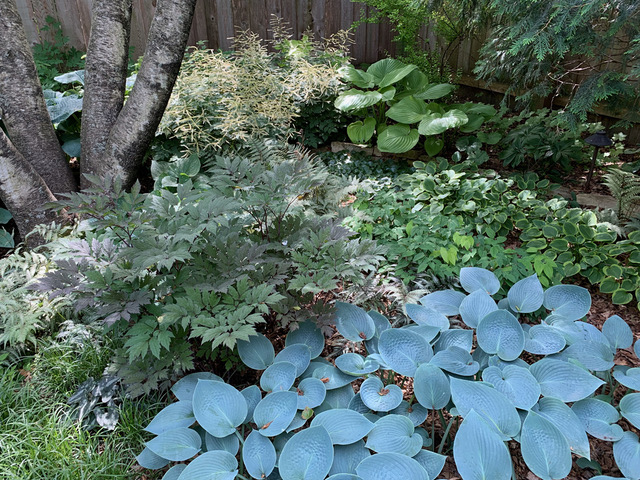This image depicts a lush backyard garden designed to mimic a forest-like atmosphere, featuring a diverse array of greenery. Dominating the scene is a large leafy plant in a bluish hue, prominently positioned in the bottom right quadrant. The garden is filled with various green plants, including tall grass, fern-like fronds, ground cover with small white-bordered leaves, and a striking plant with leaves as large as a person's head. A central tree with four distinct offshoots adds architectural interest, while the background reveals a gray wooden fence marking the property boundary and an evergreen tree providing additional shade. The sunlight filters through, casting dappled light across the scene, enhancing the rich tapestry of colors and textures in this peaceful, low-maintenance garden. Additional brick border dividers and smaller bushes in varying shades of green contribute to the garden's organized yet wild appearance, making it a calming and picturesque retreat.